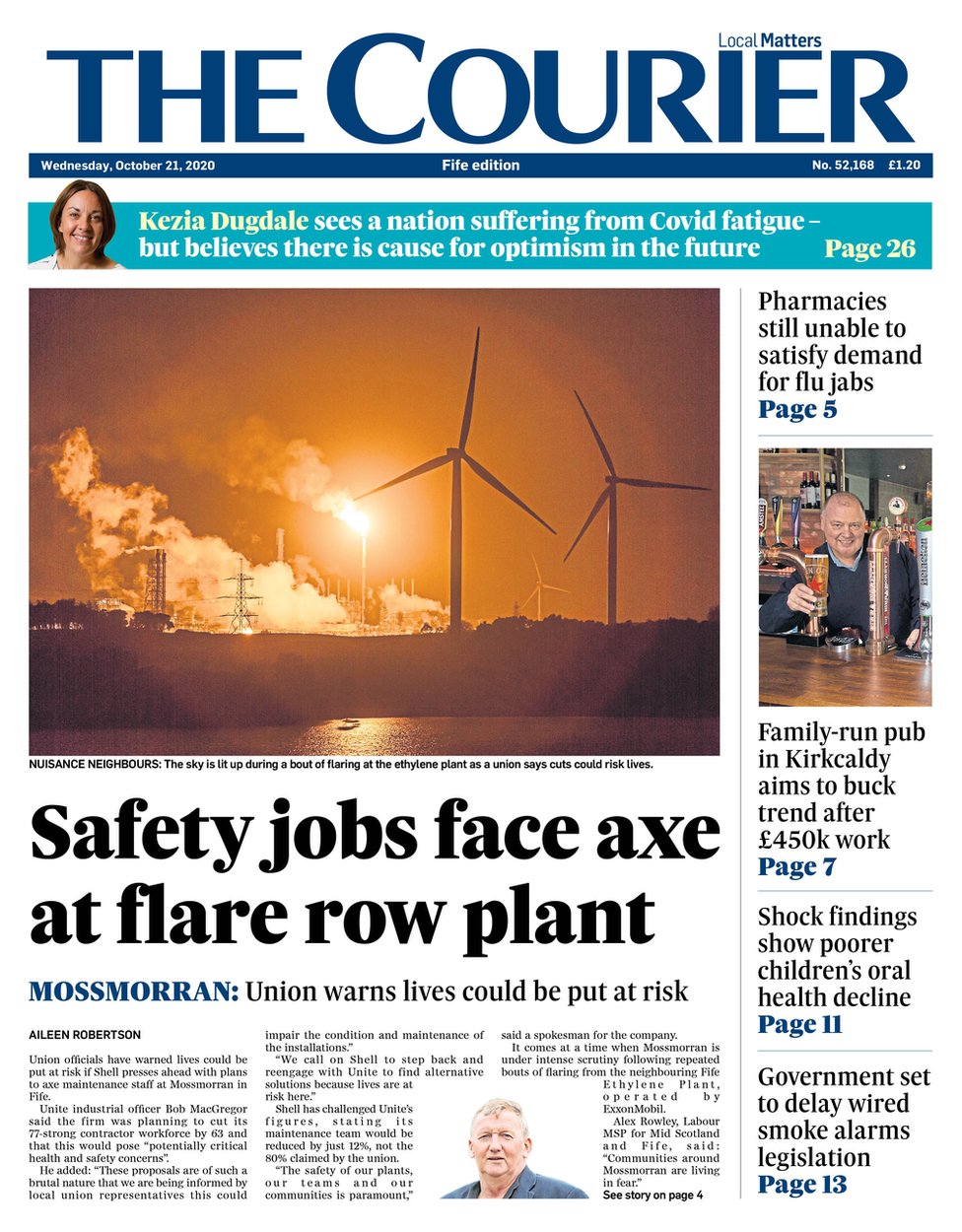**Descriptive Caption:**

This image is a screenshot of a local newspaper, titled **The Courier**, with a tagline "Local Matters" displayed over the letters "I" and "E" in the title. The title "The Courier" is written in blue at the top of the page. 

At the top left corner, the date is marked as **Wednesday, October 21, 2020**, while the center reads **Fife Edition**. On the top right, it states **No. 52.168** followed by **£1.20**.

A blue rectangular banner spans the width of the page just below the title, reading in white text: *"Kezia Dugdale sees a nation suffering from COVID fatigue but believes there is cause for optimism in the future, page 26."* To the far left within this section, there is an image of a woman presumed to be Kezia Dugdale.

Below this banner, the page is divided into several sections. To the left, there is an image of a solar plant with two windmills in the foreground against an orange and black backdrop, which includes land, water, and what appears to be emissions or smoke in the background. The caption underneath this image reads: *"Nuisance Neighbors, the sky is lit up during a bout of flaring at the ethylene plant as a union says cuts could risk lives."*

Underneath this image, there is an article titled "**Safety Jobs Space Access Flare Road Plant**" by Eileen Robertson. Accompanying this article is a picture of an unidentified man.

To the far right of the page, there are references to four different articles, including one featuring an image of a man drinking a beer at a pub.